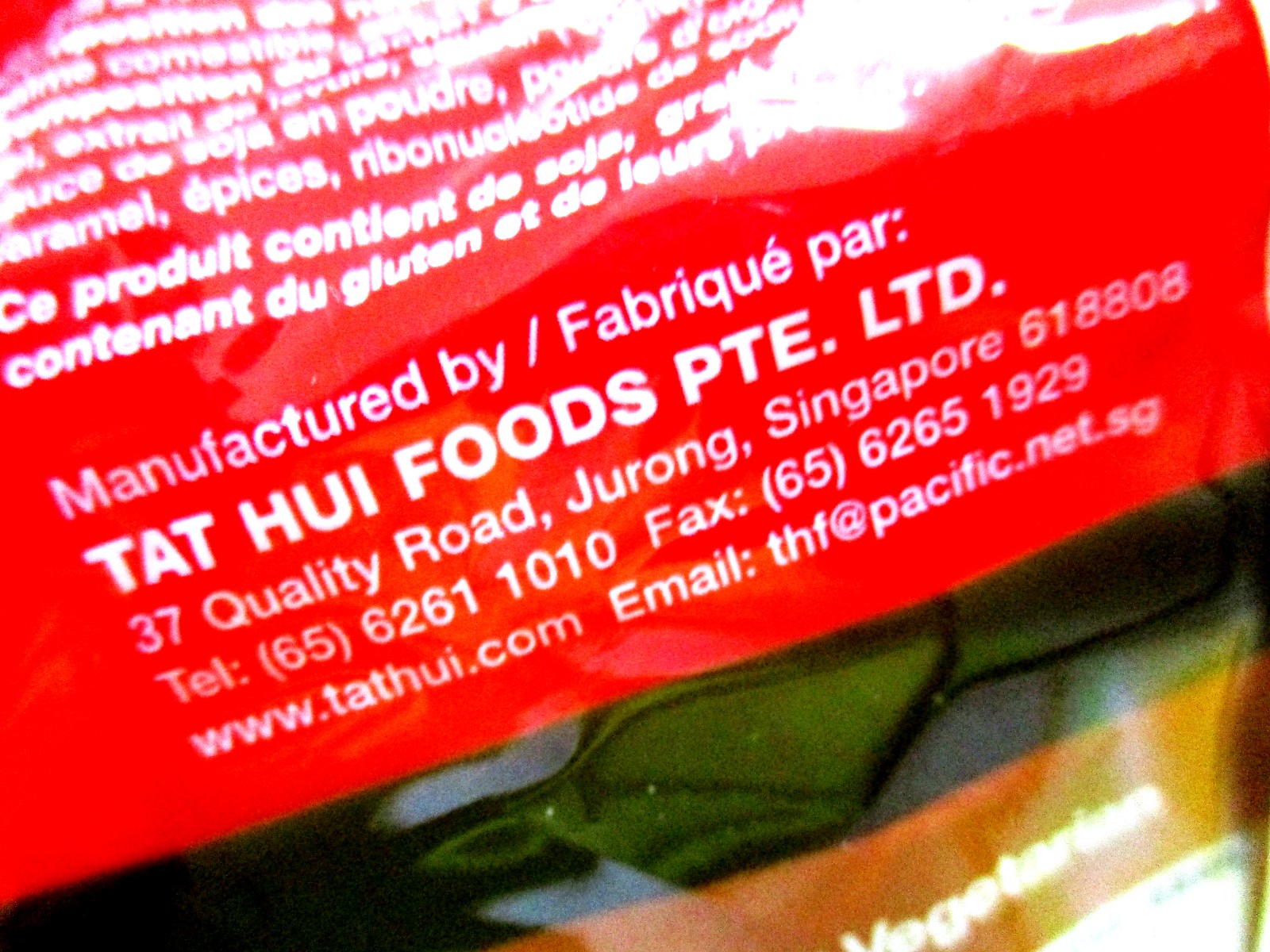The image is a close-up of a red food packaging with prominent white text details. The top section of the packaging displays "TAT HUI Foods PTE LTD" and "37 Quality Road, Jurong, Singapore 618808," indicating that it's a product from Singapore. The packaging includes a telephone number "(65) 62611010," a fax number "(65) 62651929," a website "www.tathui.com," and an email "thf@pacific.net.sg" for contact purposes. Alongside this, the text includes the word "Gluten" and mentions the content is in a different language. Below this red packaging, another product is visible with green and orange colors and the word "vegetarian" written on it. The packaging appears slightly angled and light shines off it, which makes some of the text hard to read.